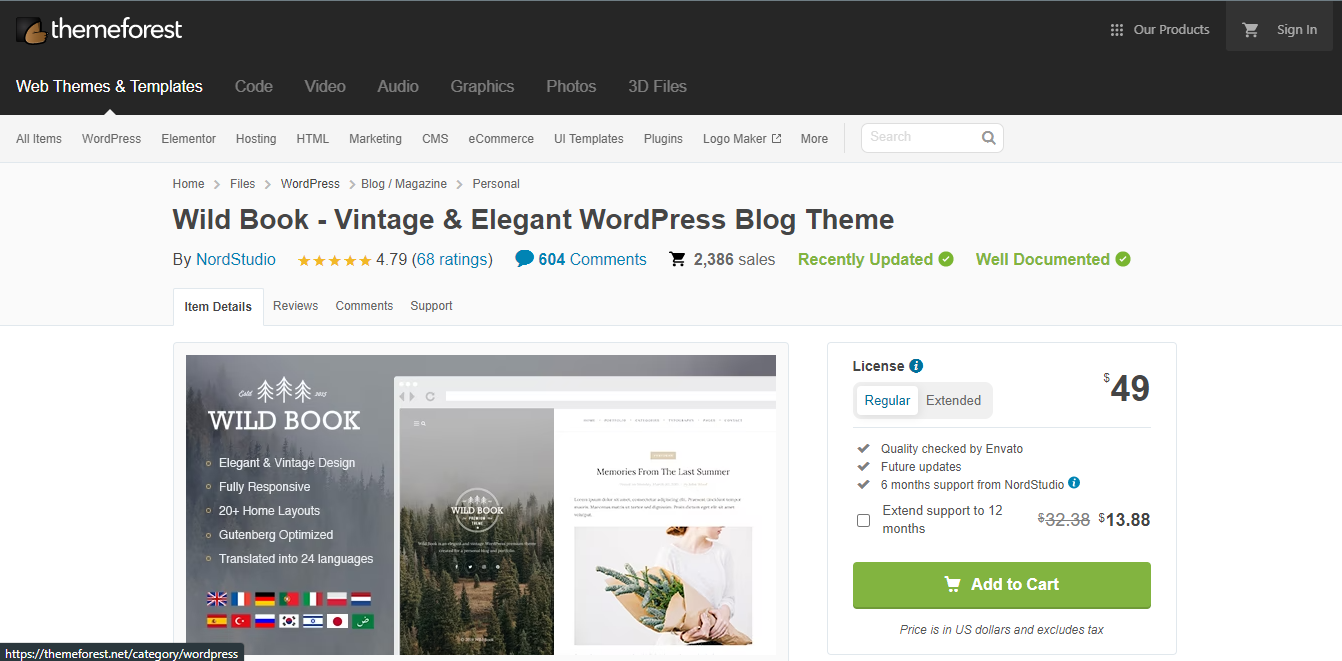Sure, here’s a cleaned-up and detailed caption for the image:

---

This is a detailed screenshot of a premium WordPress theme webpage on ThemeForest, an online marketplace for web templates and themes. At the top-right corner of the page, there are options for "Our Products" and "Sign In." The navigation bar contains seven tabs: Web Themes & Templates, Code, Video, Audio, Graphics, Photos, and 3D Files. The user is currently on the "Web Themes & Templates" tab. Below this, there is a search bar with several category options including WordPress, Elementor, Elementor Hosting, HTML, Marketing, CMS, E-commerce, UI Templates, Plugins, Logo Maker, and more.

The breadcrumb trail reads: Home > Files > WordPress > Blog/Magazine > Personal. The main content area describes the "Wild Book" — a vintage and elegant WordPress blog theme by Nord Studio. It holds a rating of 4.79 out of 68 reviews, has 608 comments, and boasts 2,386 sales. The theme is recently updated and well-documented, as indicated by check marks.

A preview image of the "Wild Book" theme shows its elegant and vintage design, mentioned to include over 20 home layouts. To the right, the license details are listed: a regular license for $49, which includes quality checks by Envato, future updates, and six months of support from Nord Studio. An optional extension for 12 months of support is available at a discounted rate of $13.88, marked down from $32.38. Below this information is an "Add to Cart" button. 

---